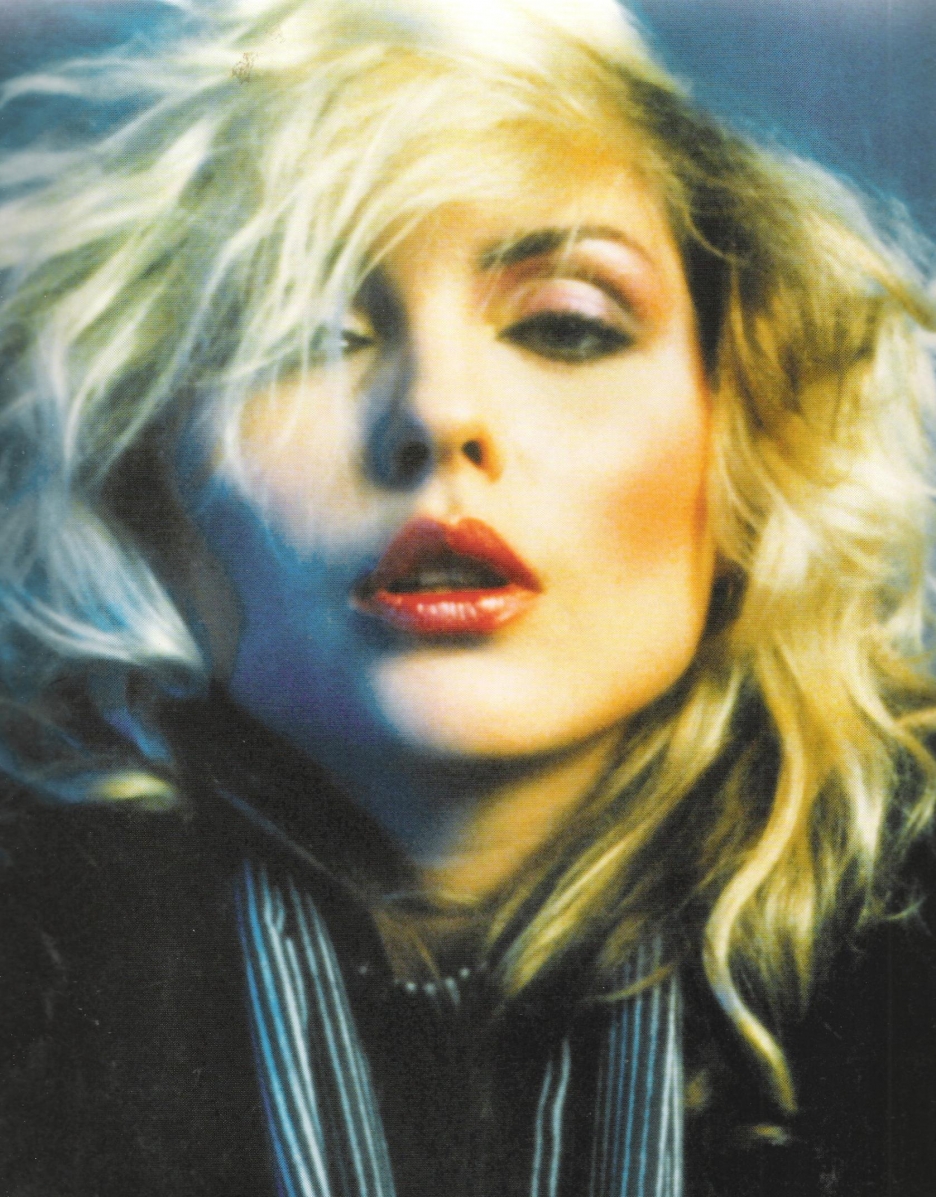This is a professionally photoshopped image of the singer Deborah Harry. She is dressed in a dark outfit with a blue, black, and white scarf elegantly wrapped around her neck, beneath a turned-up collar. Deborah's fashionably tossed, wavy blonde hair, streaked with dark roots, cascades partially over her right eye, catching the dramatic backlighting that creates dynamic highlights. Her slightly parted lips, painted a bright red, suggest she is either singing or adopting a seductive pose. Her eyes are gently closed as she gazes slightly downward at the camera. The skin tones in the image range from blue to yellow, gold, and pink, indicating a sophisticated filter application, enhancing the striking visual contrast. The focus is primarily on her face, with just a hint of the upper chest visible, capturing an iconic blend of allure and artistry.